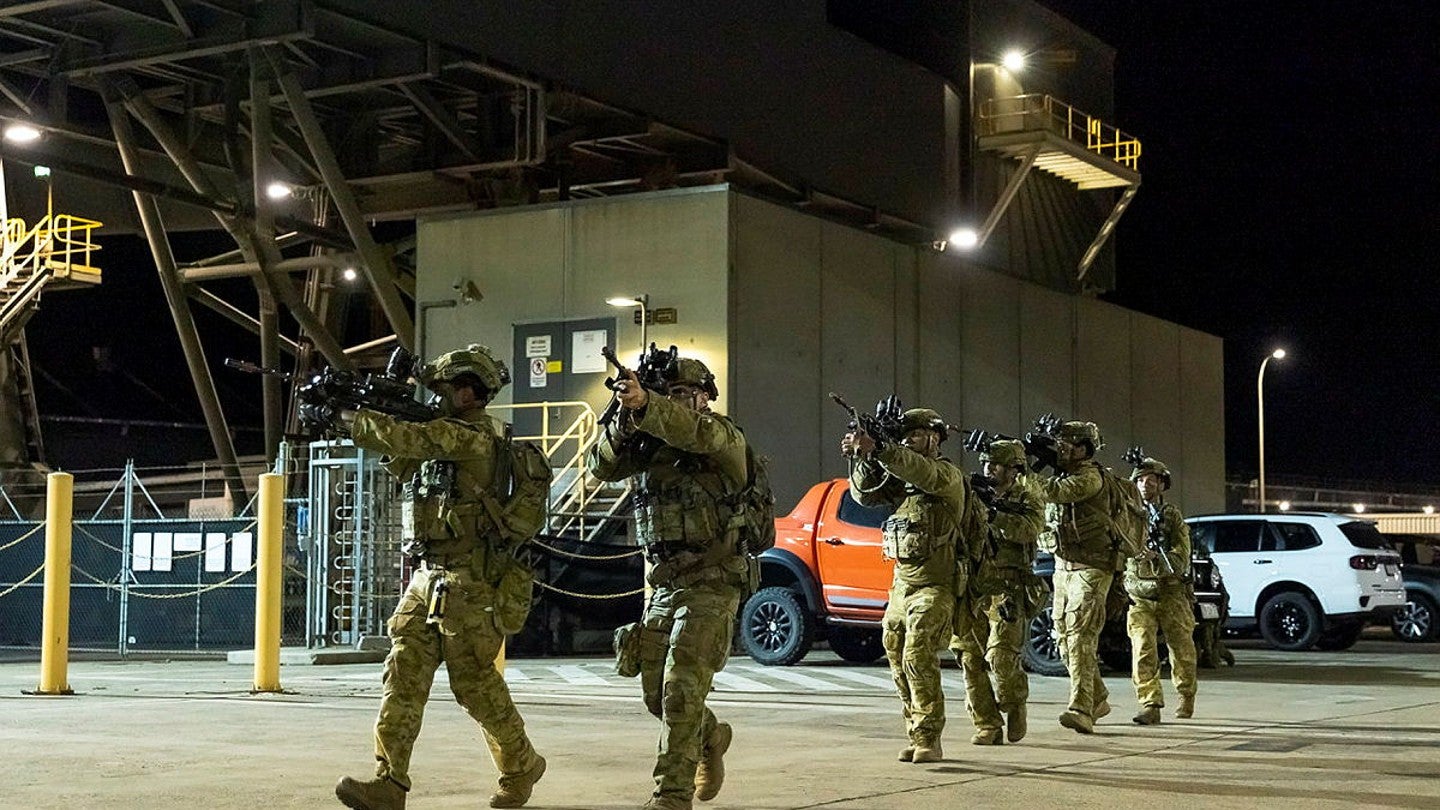In this nighttime outdoor photograph, six individuals, potentially a U.S. military unit possibly Marines, are in a parking lot, all dressed in camo military outfits with helmets and holding black guns pointed ahead. The camo features shades of green, brown, and tan. It is difficult to discern their gender, but they appear to be men. The ground is an asphalt surface marked with white lines, suggesting a parking lot. Behind the group, there are three cars: an orange one in the foreground, followed by a white car, and a darker car, possibly black. These cars have black tires and silver rims.

The background features a gray building with blue doors, adorned with signs in yellow, red, black, and white. The building includes various yellow elements: parking poles, a stairway with chains, and a raptor-like figure hanging on its side. The scene is lit with bright white lights, emphasizing the nighttime setting. Additionally, a structure with yellow posts and a closed blue gate with silver accents is present. There is also a range of equipment around, contributing to a busy, professional atmosphere—though the photo itself may not have been taken professionally.